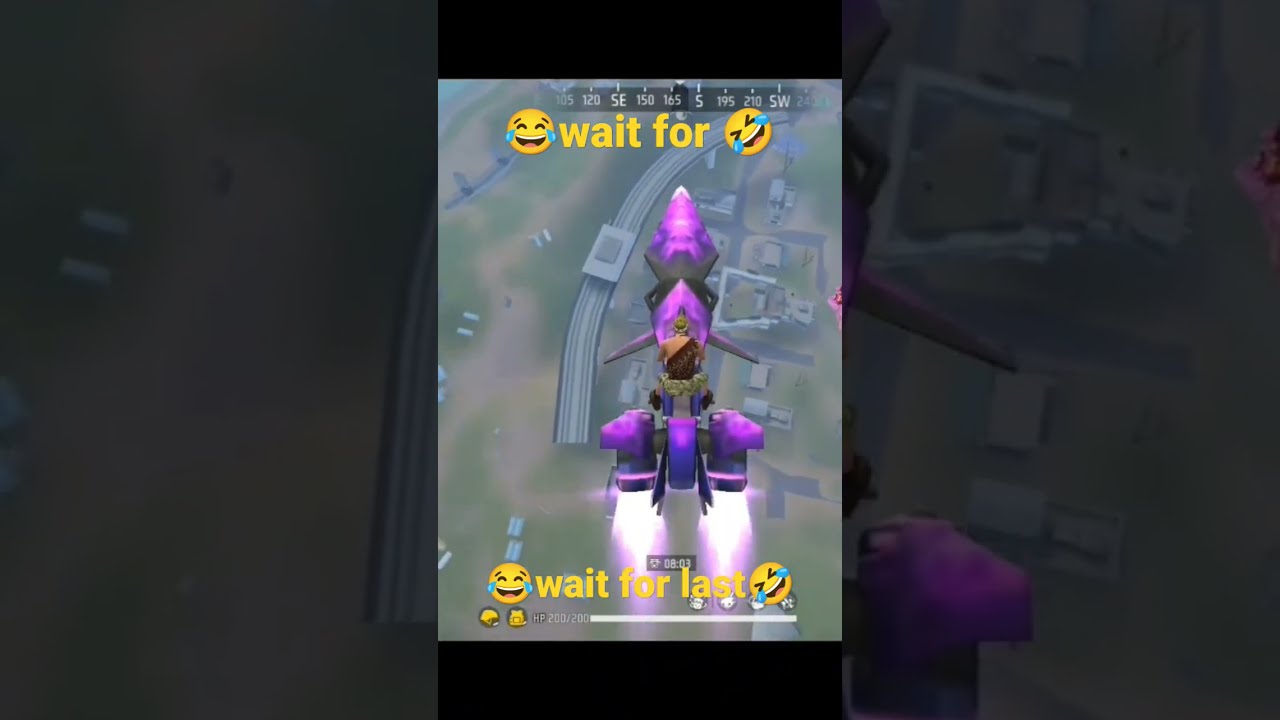The image appears to be a screen grab from a video game, likely taken on a mobile device due to the aspect ratio resembling that of a smartphone. Central to the image is a purple rocket bike, a hybrid between a rocket ship and a motorcycle, adorned with two diamond-shaped structures at the front and thin wings at their base. The bike has a central fender at the back flanked by bags that seem to house the rocket boosters propelling it through the sky. The perspective is a bird's-eye view, showing the vehicle soaring above a grayscale cityscape with visible buildings and highway networks below. Riding the rocket bike is a figure who appears to be Caucasian, wearing a green hat, camouflage pants, and a brown shirt or toga with a single strap. Overlaid on the image, in yellow font, are the words "wait for" accompanied by two crying emojis, and at the bottom, "wait for last" again flanked by two crying emojis, suggesting that the image is part of a humorous meme where something funny is anticipated to happen. Additionally, a compass is seen at the top of the image, indicating a south-southeast direction, and the image includes some darker, enlarged sections of the ground on the left and right sides, framing the central action.